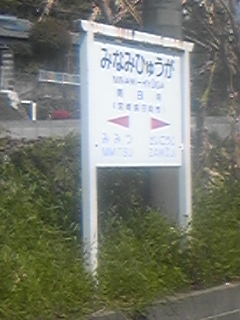This image is a hazy, blurry photograph of a directional sign in a foreign language, likely Japanese or Korean. The sign, which is white and wooden, is situated in front of a building, possibly a brick one, and stands on a slight hill or slope. The sign is perched amongst natural vegetation, including low-to-the-ground shrubbery and tall grasses, transitioning to shorter grass as it nears a small gray wall at the base. The sign itself features multiple lines of black text, consisting of a large heading with approximately eight bold Asian characters, followed by more lines of smaller text. This text appears exclusively in Asian characters, with none in English. Below these lines of text are two red arrows, one pointing to the left and the other to the right, each accompanied by additional characters that likely describe destinations or directions. The sign is mounted on tall posts and is angled diagonally, facing slightly to the right from the viewer's perspective. In the backdrop, various buildings are visible beyond the vegetation.